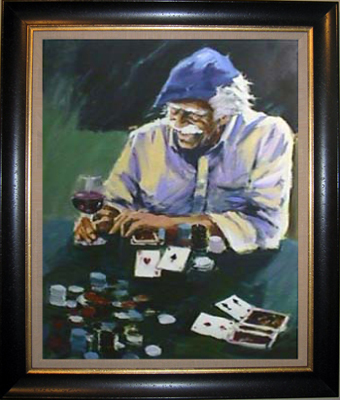The image features an oil painting encased in a double-layered frame. The outer frame is polished black lacquer, raised in the center, measuring about a quarter of an inch in width and reflecting light. There is a thin strip of gold inside the black frame, followed by a thicker, flat gray mat that surrounds the painting itself. The background of the overall painting is plain white. 

The composition captures an older gentleman, potentially African American, seated at a green poker table. The man, seen from the chest up, has gray hair, gray eyebrows, and a thick gray mustache. He dons a royal blue hat and a button-down shirt with rolled-up sleeves, detailed in yellow and blue hues with a collar. In his right hand, he holds a glass of red wine.

In front of him on the table lay two aces among an array of poker chips and scattered cards, possibly hinting at a game of blackjack. The painting is characterized by slightly blurry details and an abstract texture, particularly noticeable on the shirt, indicative of the oil medium used. The setting evokes a relaxed, contemplative moment in the midst of a poker game.